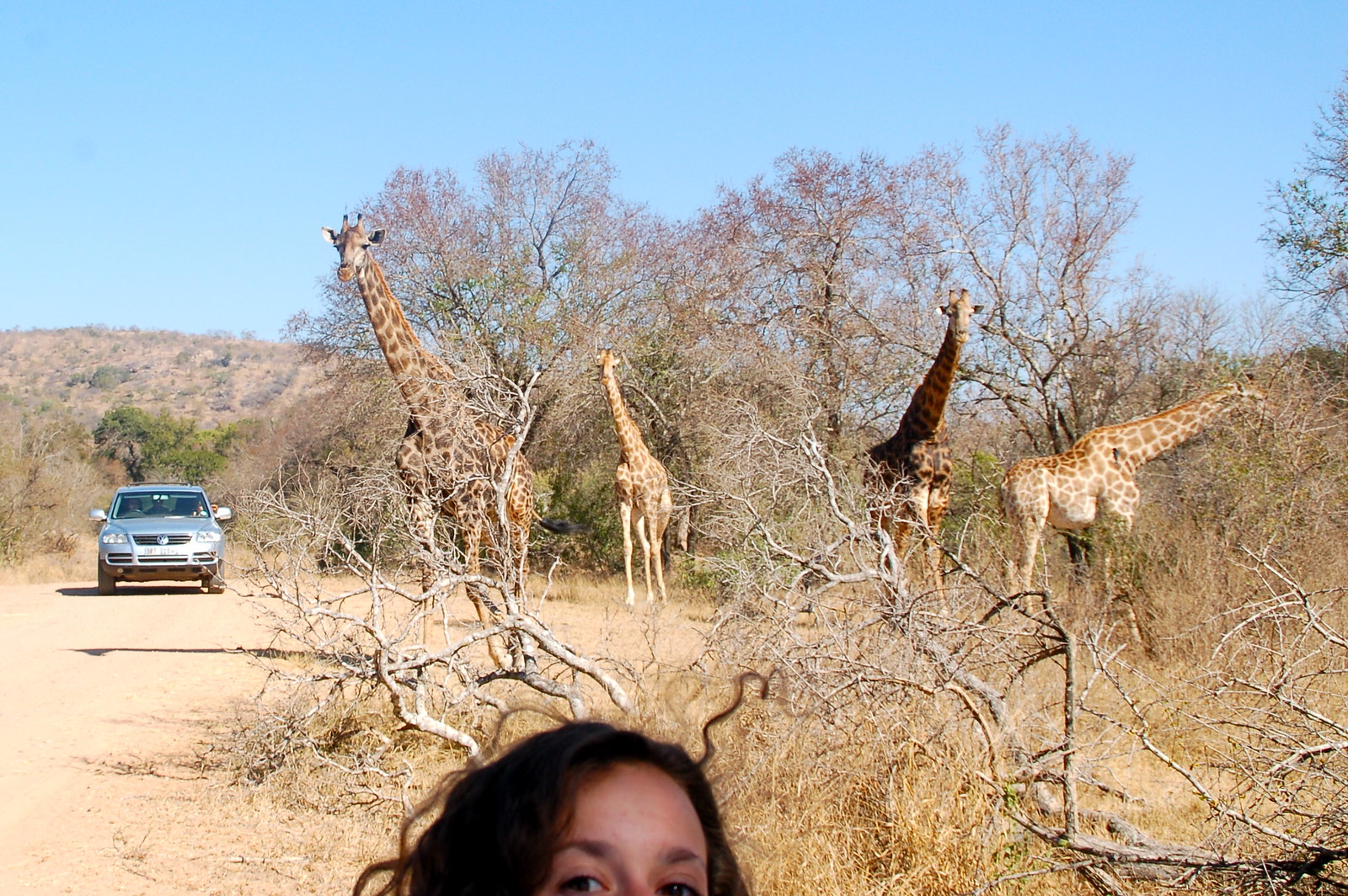In this captivating photograph, a serene safari scene unfolds under a clear blue sky. In the forefront, partially obscured but unmistakably curious, a young girl with tan skin, dark eyes, and long brown hair gazes towards the camera, only her eyes and the top of her head visible, as though she's taking a selfie. Surrounding her, a dry clearing stretches out, scattered with light brown and gray dead trees and sparse brush in shades of brown and yellow. To the left side of the frame, a silver SUV with a gray underside is parked on a dirt road, seemingly on a family outing. The vehicle is bordered by a hill in the distance, mostly brown and gray but dotted with sparse green plants and a few evergreen trees with lush green leaves. Center stage, a majestic group of giraffes stands tall against the rugged landscape. Their tan coats adorned with chocolate brown spots, these gentle giants include two adults, one juvenile, and a baby. While three face the camera, the fourth giraffe, in profile, stretches its long neck to nibble from the brush, highlighting the rich diversity of life in this wild and arid panorama.